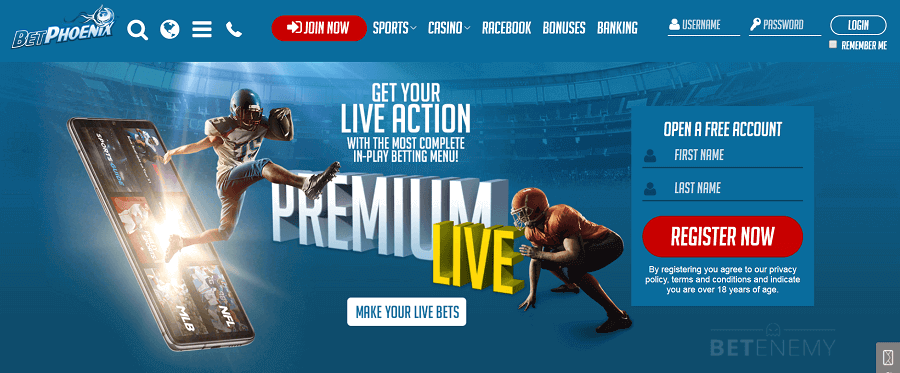The image features a predominantly blue webpage for BetPhoenix, showcased in the upper left corner with the text "BetPhoenix" followed by a search magnifying glass icon, a globe icon, a three-line menu icon, and a call icon. A prominent red button labeled "Join Now" is located near the top.

The interface displays several dropdown menus labeled "Sports," "Casino," "Racebook," "Bonuses," and "Banking," followed by entry fields for "Username" and "Password" with a checkbox for "Remember Me." A login button is situated nearby. 

The background is a photograph of a stadium bathed in dark blue and teal tones. Centered prominently is an American football player leaping out from a cellphone screen, clutching a football, while another player is in a crouched position on the ground, supporting himself with one hand. 

Text in white reads, "Get your live action with the most complete in-play betting menu, Premium Live," with "live" highlighted in yellow. A clickable button labeled "Make Your Live Bets" is shown, alongside an invitation to "Open a free account" with fields for "First Name" and "Last Name," and a red "Register Now" button. A disclaimer informs users that by registering, they agree to the privacy policy and terms and conditions and confirm they are over 18 years of age. 

At the bottom right corner, the text "BetEnemy" is visible.